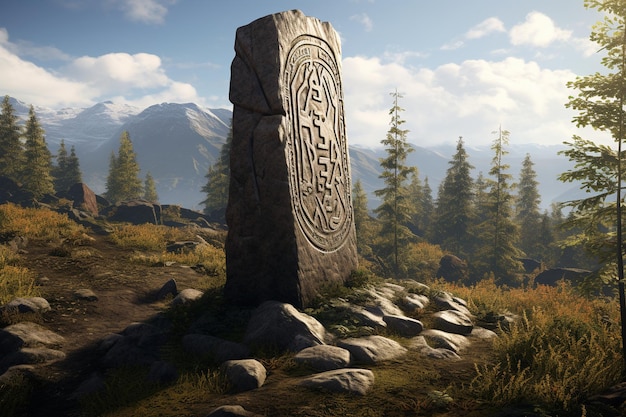The image portrays an AI-generated, highly detailed scene of a mountainous region featuring an ancient artifact. At the center of a ground area stands a large stone monolith that is almost cuboidal but not perfectly shaped, and green in color with an abstract design resembling a map or deity carved into its surface. This structure, possibly a stela or ancient signpost, is positioned upright, surrounded by smaller stones and patches of green and yellowish grass. A trail runs beside the monolith, suggesting its historical role as a guidepost. Further away, the ground transitions into a dense array of green trees, typical of pine, that frame the open clearing. In the background, majestic snow-covered mountains rise high under a sky filled with both white clouds and patches of blue. The overall setting on an elevated hill creates an aura of ancient mystery within this richly detailed, natural landscape.